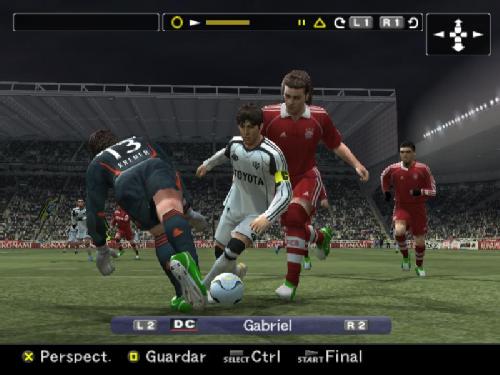In this screen capture of an advanced soccer-themed computer game, the scene showcases a highly detailed and animated match on a lush green field. At the forefront, there are two players dressed in red jerseys sprinting toward the viewer. One of these players is closing in on a player in white, who is also facing the viewer and appears ready to kick the ball. A player in black, with his back turned to the viewer, is also in pursuit of the ball.

The game interface includes a bar at the bottom displaying "DC Gabriel," possibly indicative of the character being controlled or a specific game mode. In the background, more animated player characters are scattered across the field, actively engaged in the match. Further in the distance, the grand stand is filled with a lively crowd, and above them, the edge of a stadium roof arches under the dark expanse of a nighttime sky, adding to the immersive atmosphere of the game.